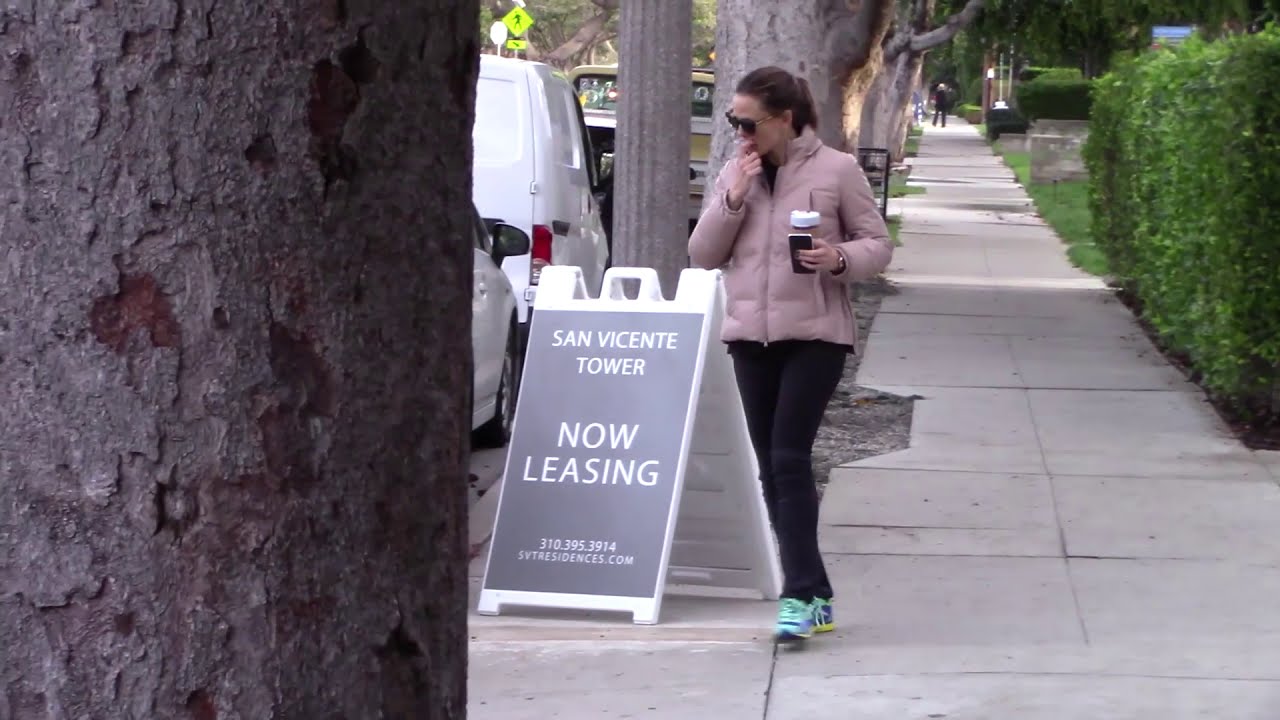In this detailed image, a woman stands on a tree-lined sidewalk holding a coffee cup and a cell phone in her left hand. She is clad in a pink puffy coat, likely indicating chilly weather, paired with blue jogging pants and turquoise running shoes. Her dark hair is pulled back into a ponytail, and she wears sunglasses, with her right hand raised to her mouth, possibly taking a bite of something. Adjacent to her, a large tree trunk dominates the left third of the image, and next to it, a sign reads "San Vicente Tower Now Leasing" with a phone number and contact information. The backdrop includes several vehicles and well-tended bushes, with additional homes visible on the right. The sidewalk itself is in moderate repair, showing some cracks and missing pieces. Farther down, another person can be faintly seen in the distance.